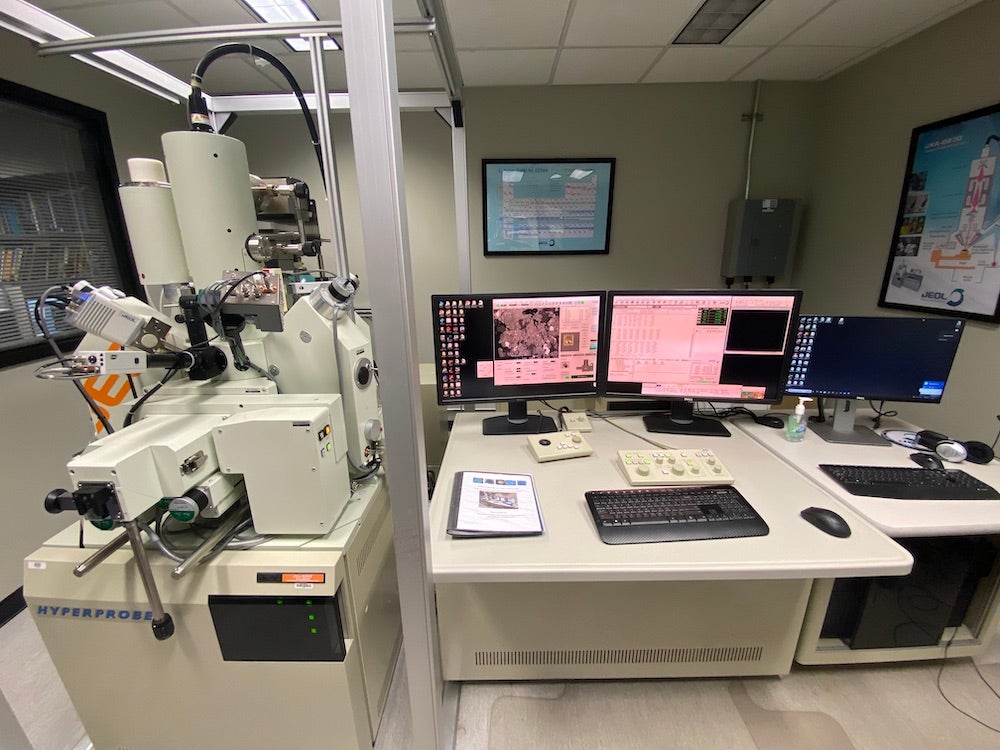This image is a detailed color photograph of an office that appears to be part of a medical office or science lab. The room features gray walls adorned with several indistinct black-framed pictures and diagrams. Prominently displayed in the middle of the image is a white desk situated on the right side, hosting two black computer monitors showing pink screens, a black keyboard, and a black mouse. There are also some white horizontal control units with knobs, likely connected to the adjacent machinery.

To the right of this, another smaller white desk holds a monitor with a black screen, another black keyboard, a black mouse, and a bottle of hand sanitizer. The left side of the image showcases an advanced piece of scientific or medical diagnostic equipment branded "HyperProbe." This machine, beige in color, consists of a large rectangular base standing about three feet, with multiple white cylinders and numerous cables connected to it.

A rectangular binder with a clear cover containing a white sheet of paper also rests on the main desk. Additional details include a window on the left wall peering into an adjacent room, a circuit breaker box on the back right wall, synthetic hardwood flooring, and a ceiling composed of Styrofoam tiles supported by gray plastic. The entire space is well-lit by fluorescent lighting.